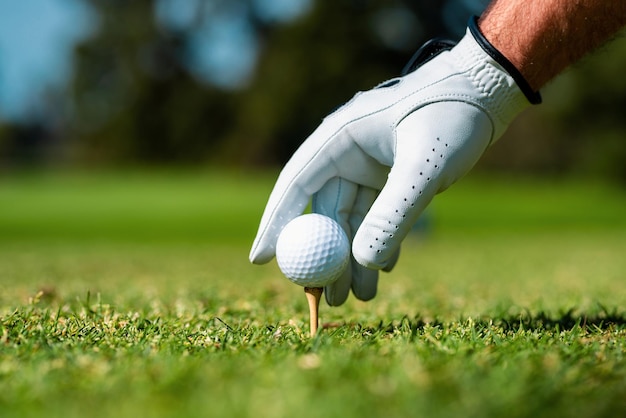In this detailed photograph of a golf course, the foreground features blurred, well-maintained green grass with slight hints of yellow. At the center, a man's right hand adorned in a skin-tight white leather golf glove with small ventilation holes, and black trim around the wrist, reaches down from the upper right corner. This gloved hand, displaying the man's lightly hairy forearm, is in the act of placing a dimpled white golf ball onto a beige wooden tee embedded in the short grass. The background blurs into a tree line with dark green silhouettes and a patch of light blue sky peeking through the upper left corner, adding depth and a sense of calm to the scene.